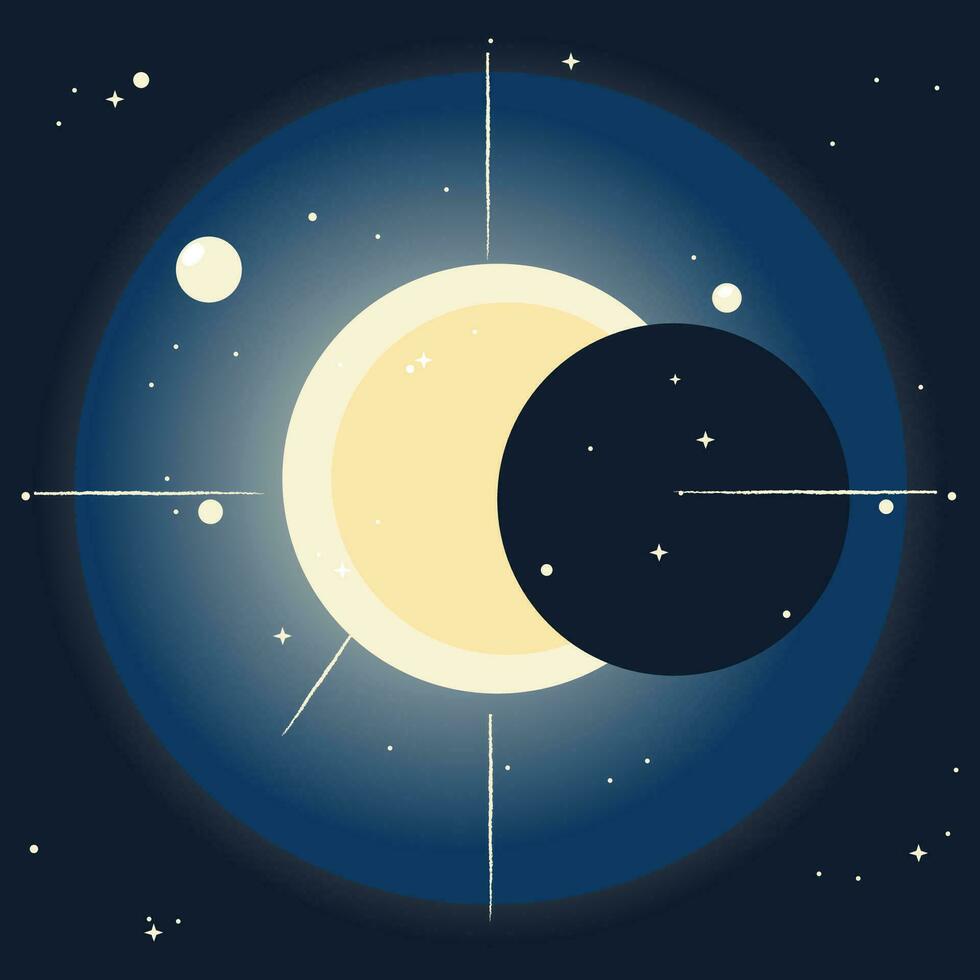This painting depicts an outer space scene with a black background, filled with varying sizes of stars and dots that create a cosmic ambience. Dominating the center is a large blue circular shape, reminiscent of a car tire in thickness, with lighter shadings of blue blending through it. Inside this blue circle, a white circle with yellow in its center is embedded, resembling a glowing sun or planet. To the right of this central yellow and white sphere, there is a smaller black circle, possibly suggesting an eclipse, which also contains stars within it. The composition is crisscrossed by white lines: a vertical line runs from the top to the bottom of the blue outer circle, intersecting the central yellow sphere, while horizontal lines extend from the left to the right side of the canvas. Additionally, a smaller diagonal line extends towards the lower left corner from the central yellow sphere. The arrangement of the circles and intersecting lines against the star-studded background gives the artwork an eye-like appearance when viewed from a distance.